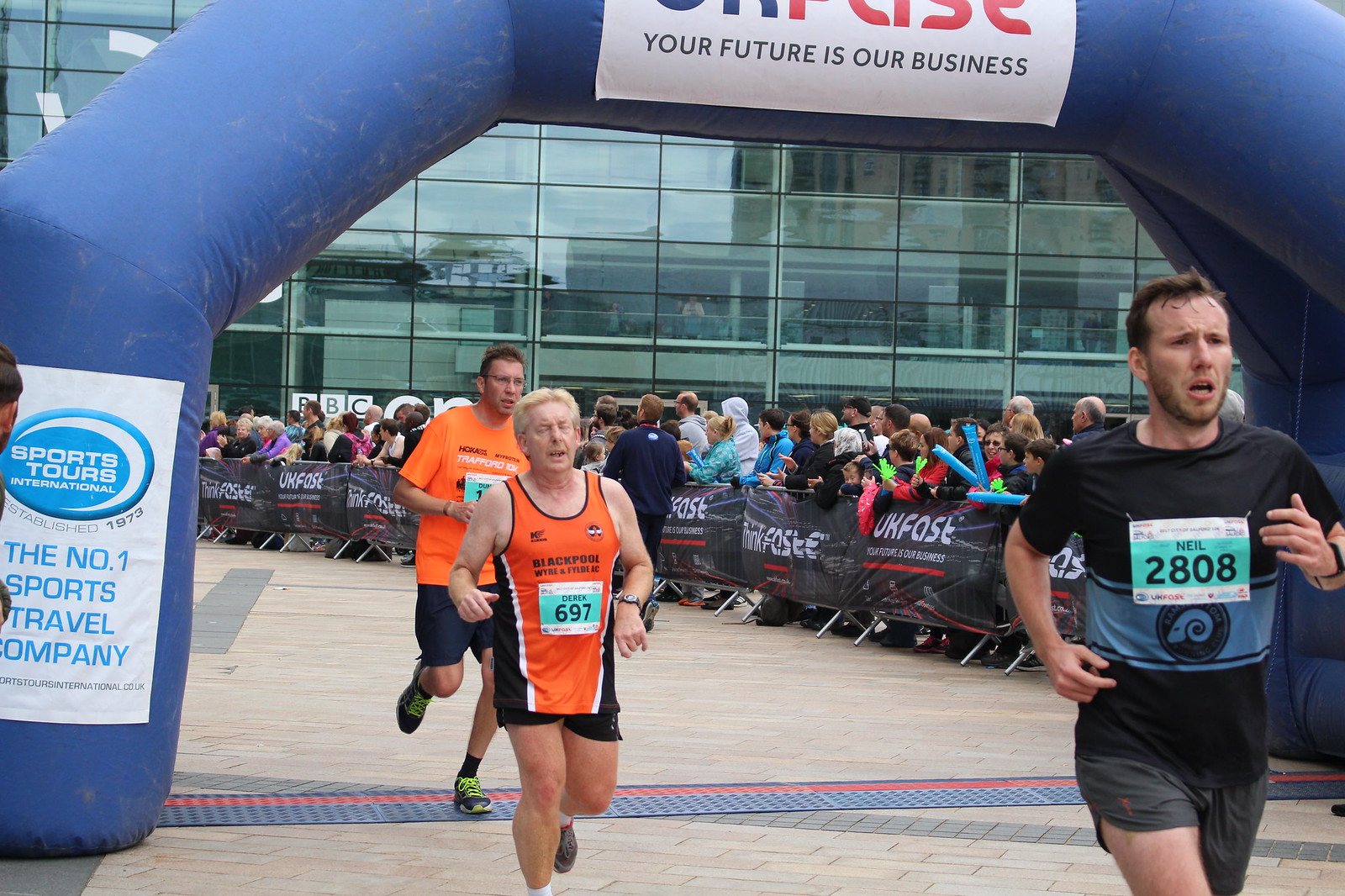In the image, we see the culmination of a foot race on a brick runway, captured during the middle of the day. The scene is bustling with activity, featuring three male runners approaching the finish line, which is dominated by a large inflatable arch adorned with sponsorship logos. The arch, emblazoned with the phrase "Your Future is Our Business," marks the end of the race. 

The man in the foreground, wearing the number 2808, and another runner beside him, number 697, have already crossed the finish line. A third runner is just stepping over the threshold, although his race number is obscured. The energetic atmosphere is heightened by a crowd of spectators gathered behind metal barricades on the right side of the frame, enthusiastically observing the scene.

The setting is an outdoor venue with a building visible in the background. The vivid colors in the image—blue, white, dark blue, red, light blue, orange, pink, green, and light green—enhance the lively and dynamic feel of the event.